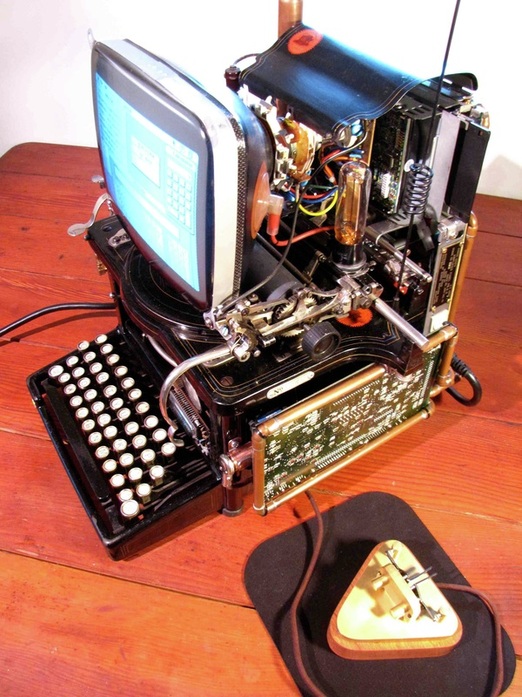The image portrays a scene with an almost ancient, homemade computer-like machine resting on a wooden table with slats. The background is a plain white wall, which emphasizes the machine's intricate and exposed design. The contraption features a small, blue screen with a white border, facing the left, and a circular-keyed keyboard reminiscent of an old typewriter strapped below the screen. A unique, triangular mouse is situated to the far right, complete with visible cables and potentially electrodes, connected to the unexplained device. The entire setup exudes a raw, mechanical aura, with all internal components such as wires, springs, and various colored circuitry (including black, silver, red, yellow, and blue) laid bare. This makeshift computer is a fusion of retro elements and raw mechanics, giving it a distinct, primitive appearance.